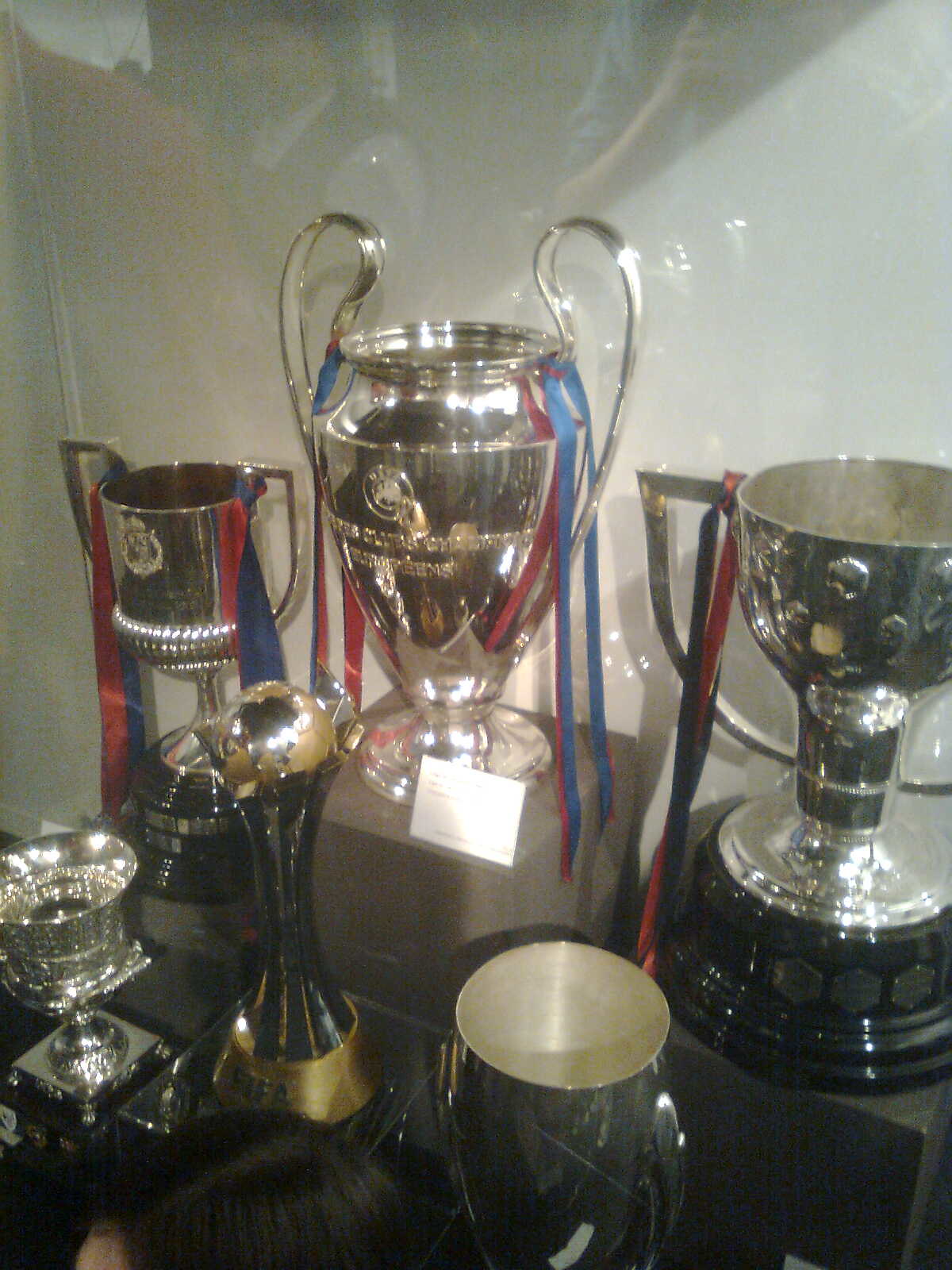The image features a display of six silver trophies encased behind a glass case with a reflective white background. Three of the larger trophies prominently positioned in the back have large, elaborate handles on both sides and are adorned with colored streamers, mainly in blue and red, which likely suggest affiliations with European football clubs such as Barcelona or Bayern Munich. The leftmost trophy has multiple handles with a thick navy and red streamer on each side, while the central trophy has notable blue and red streamers hanging from its handles.

In the foreground sit smaller silver trophies, also cups, but without the large handles. One of these trophies features intricate engraved designs and is situated on a small brown block. Another notable piece among the trophies is a distinct gold and black trophy in the center of the display, showcasing a golden base, a black, elongated neck, and a gold and black spherical design at the top, possibly emblematic of a unique award style.

There is also a woman partially visible in the foreground with black hair parted in the middle. These trophies rest on a dark brown table that supports their varied elevations with smaller brown blocks. Alongside the trophies, one can also identify the UEFA emblem and inscriptions denoting club championships, from the prestigious Champions League cups to possibly equivalent European titles.